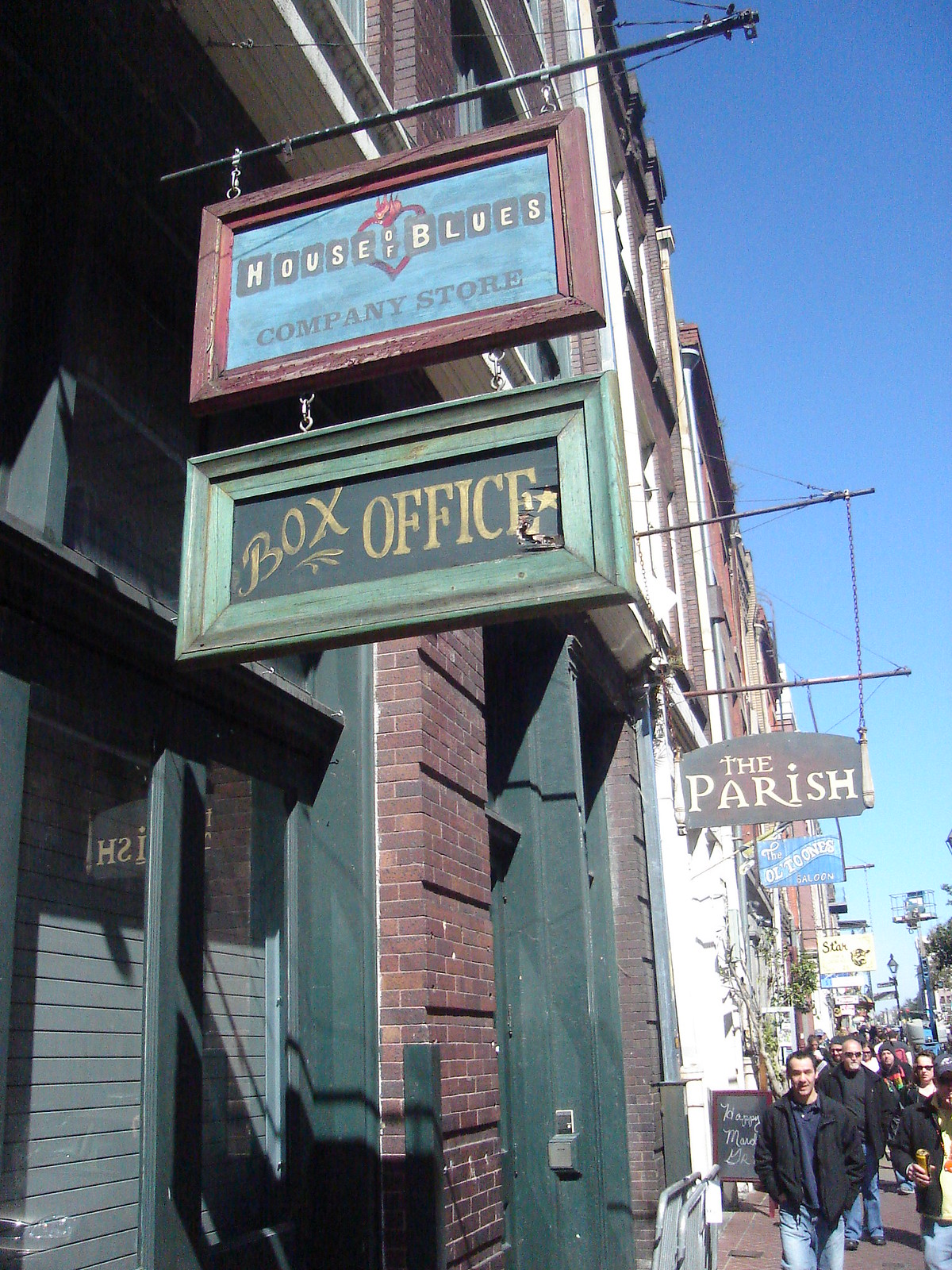This image captures a bustling downtown scene, seemingly outside a pub or similar venue. The focal point is the House of Blues Company Store and its box office, indicated by two hanging signs connected via a chain. Further down on the right, another business, The Parish, displays its sign. The street is alive with pedestrians, many of whom are men in jackets, suggesting a chilly yet sunny day. The bright blue sky overhead contrasts with the timeless charm of the brick buildings lining the street, characterized by green-painted windows and doorways. In the distance, additional signs hint at more businesses, though their details fade with the street's length. The vibrant interplay of sunlight and the crowd's energy conveys a lively atmosphere in this historic part of town.